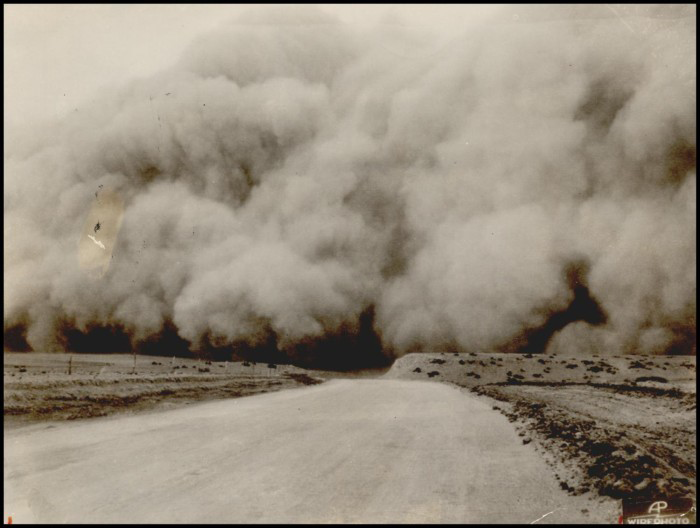This old black and white photo from the Great Depression-era, possibly from the 1930s Dust Bowl, is eerily impressive and detailed in its composition. The square photo, bordered in black, portrays a packed dirt road running from the foreground into the horizon. On both sides of the road lies flat, possibly agricultural land that looks dry, with a few clumps of dirt scattered about. Above this barren landscape, the sky is consumed by a massive, boiling cloud of dust and smoke, predominantly black at the bottom transitioning to billowing white smoke towards the top. The scene is dominated by this tumultuous cloud, giving an impression of an impending dust storm. In the upper left corner, there’s a slight break in the smoke, revealing a light gray patch. The overall sepia tone of the image enhances its dark, spooky, and ominous atmosphere. Notably, the lower right corner of the photograph bears a logo inscribed with "Wide Photo," featuring an interlinked "P" and "A."